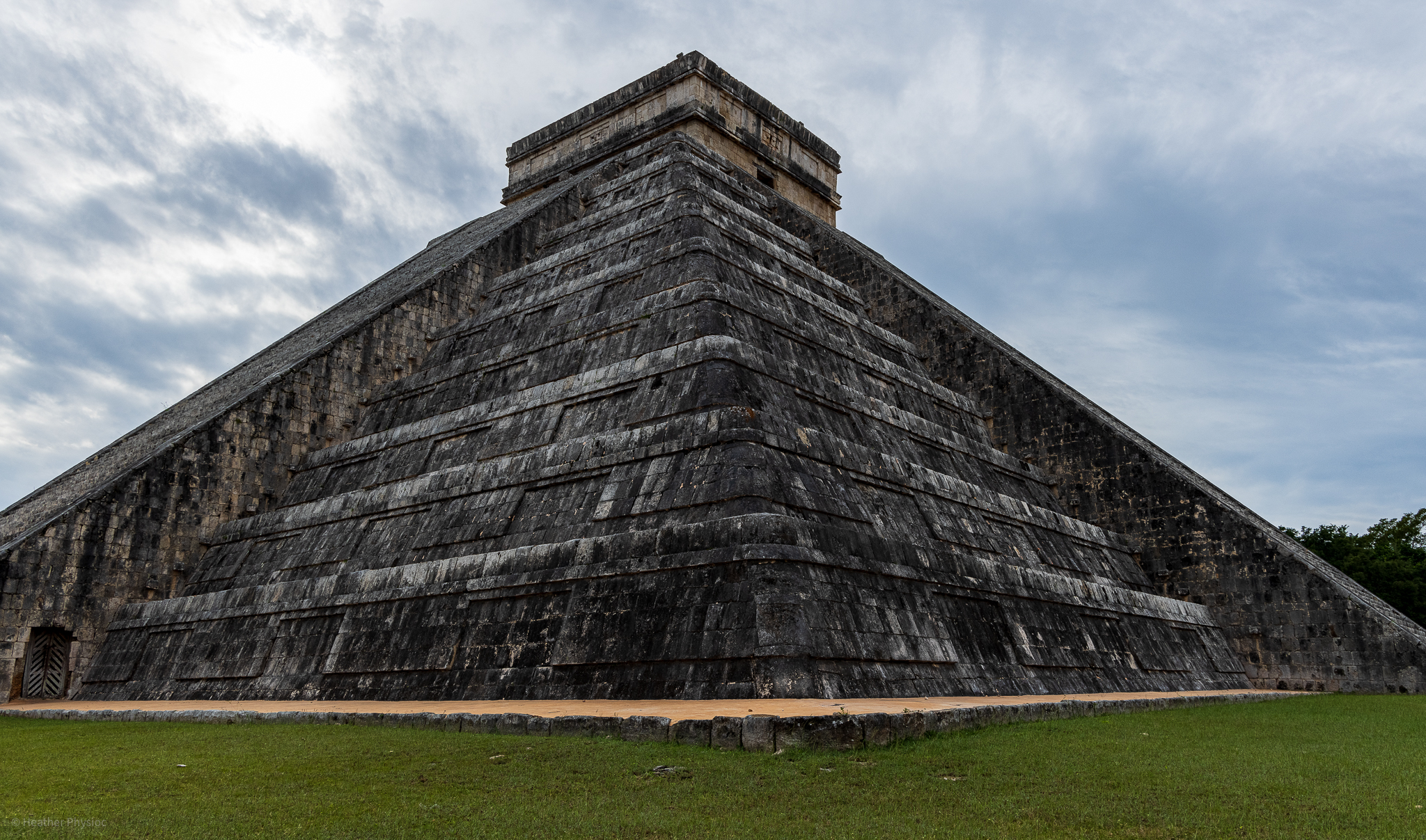This photograph captures a striking South American step pyramid, likely of Aztec or Mayan origin, distinguished by its unique architectural features. Unlike the smooth, pointed pyramids of Egypt, this pyramid is composed of several stepped terraces leading to a broad, flat platform at the top. Each of its four sides is adorned with a staircase, suggesting a place of ceremonial importance. The ancient structure, possibly used for ritual human sacrifices or other sacred purposes, shows significant weathering; its once-brown or tan stonework now stained to dark hues, likely from years of exposure to the elements. 

The image is framed with a cloudy sky that provides diffuse and even lighting, emphasizing the pyramid's aged and eroded facade. In the foreground, a manicured green lawn contrasts sharply with the structure's dark, worn stone. An orange-salmon colored walkway encircles the pyramid, further highlighting its majestic yet somber presence. On the right, behind the pyramid, trees can be spotted, adding to the sense of an ancient ruin situated within a natural landscape.